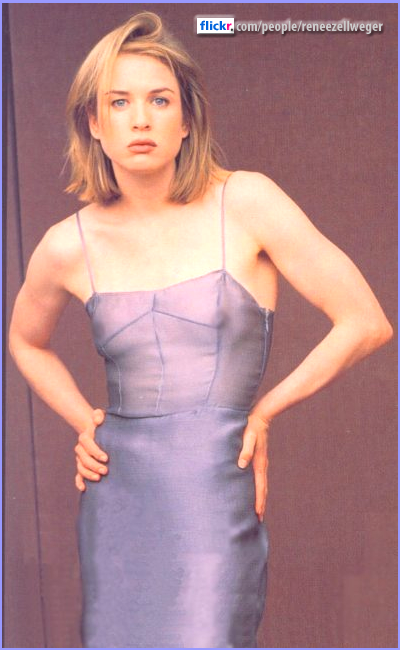The image features a young Renée Zellweger standing against a textured, brownish-purple background with a slightly darker purple line running downward on the left side. In the upper right corner, a white box displays "Flickr," with blue text for "flick" and a red "R," followed by "flickr.com/people/Renée Zellweger" in white text. Renée, wearing a form-fitting light blue dress with spaghetti straps, poses facing the camera with a serious expression. Her slender build is accentuated by the dress, and she holds her hands at her waist with elbows bent at about 90 degrees. Her shoulder-length brown hair, slightly tousled at the front, partially covers her face. Her striking blue eyes and full lips contribute to her overall graceful appearance.